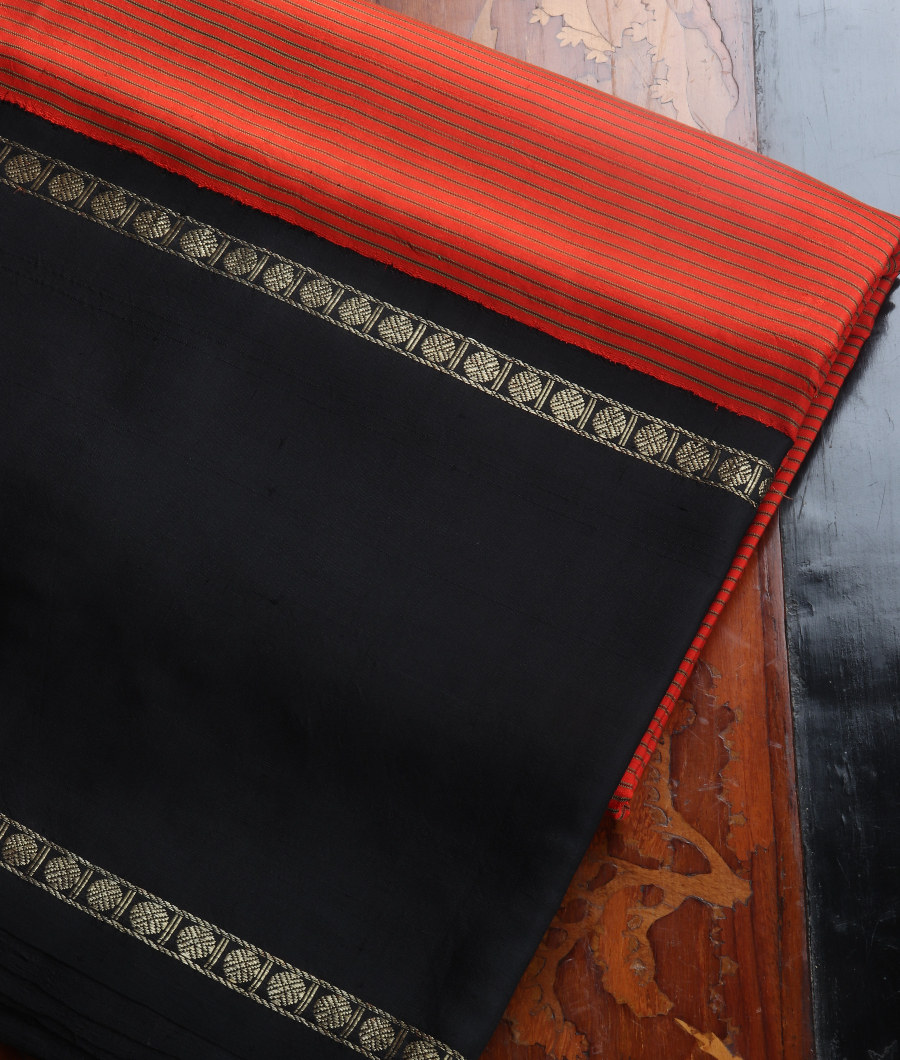The image depicts a piece of fabric with a detailed design, displayed on a weathered wooden table with a hint of black leather accents. The fabric is divided into two sections: the first section is a red cloth with thin, horizontal black stripes that resemble bookbinding edges. This section transitions into a black fabric that features horizontally aligned silver lines, bordered by golden emblems arranged in small squares. Each emblem measures about an inch to an inch and a half in height. The wood surface beneath the fabric appears aged and carries visible grain with some black ornamental details around the edges. The combination of the sharp, new-looking fabric against the worn wood creates a striking contrast.